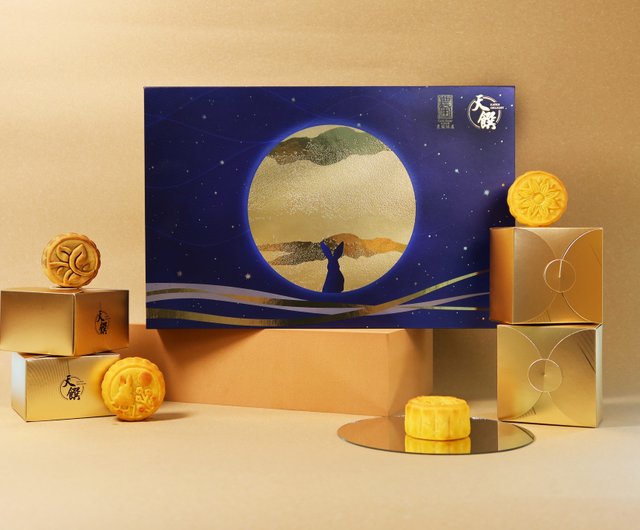The image showcases an exquisite arrangement of mooncakes displayed against a luxurious gold-like background. The setting includes a series of gold boxes, with the mooncakes meticulously positioned on and around them. Each mooncake, adorned with intricate imprints akin to those found on designer cookies such as Oreos, flaunts detailed designs of elements like sunflowers and trees. The mooncakes are notably thick and sit elegantly on reflective surfaces, adding to the sophisticated presentation.

At the center of this arrangement is a prominent, vibrant purple box featuring a large gold circle. Within this circle, a green cloud motif frames the silhouette of a rabbit, evoking imagery of the night sky. The background further accentuates this celestial theme, resembling a serene nocturnal landscape. The gold circle object, possibly a mirror, appears central and crucial to the aesthetic of the display, which carries an aura of opulence indicative of a high-end food product advertisement. This meticulously crafted scene, enriched with Japanese lettering in the upper right corner, emphasizes the luxurious and artistic nature of the mooncakes being showcased.